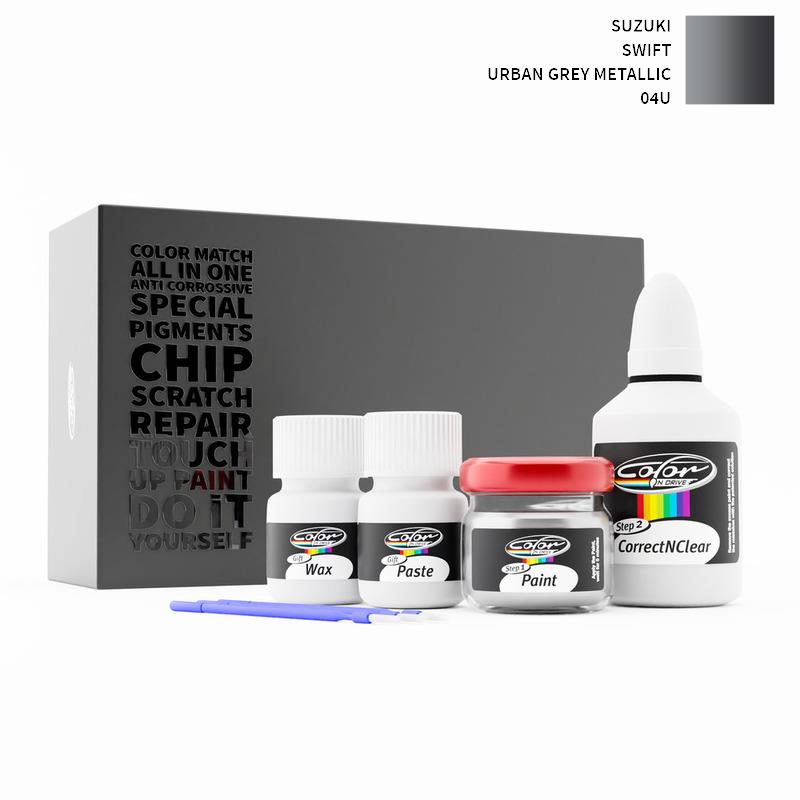The image showcases a collection of paint repair products arranged in front of a gray box labeled "Color Match All-in-One Anti-Corrosive Special Pigments, Chip Scratch Repair, Touch-Up Paint, Do-It-Yourself." The centerpiece includes four white bottles prominently displaying black labels with the brand "Color in Drive." These bottles are sequentially labeled "Color Wax," "Color Paste," "Color Paint," in a glass jar with a red screw-off lid, and a larger plastic bottle labeled "Step Two Correct and Clear." Each product features a distinct label with a sideways rainbow pattern. Additionally, small blue paint brushes with white bristles are arranged in front of the bottles. In the top right corner of the gray box, a smaller square indicates "Suzuki Swift Urban Gray Metallic, 04U," offering further color matching information.